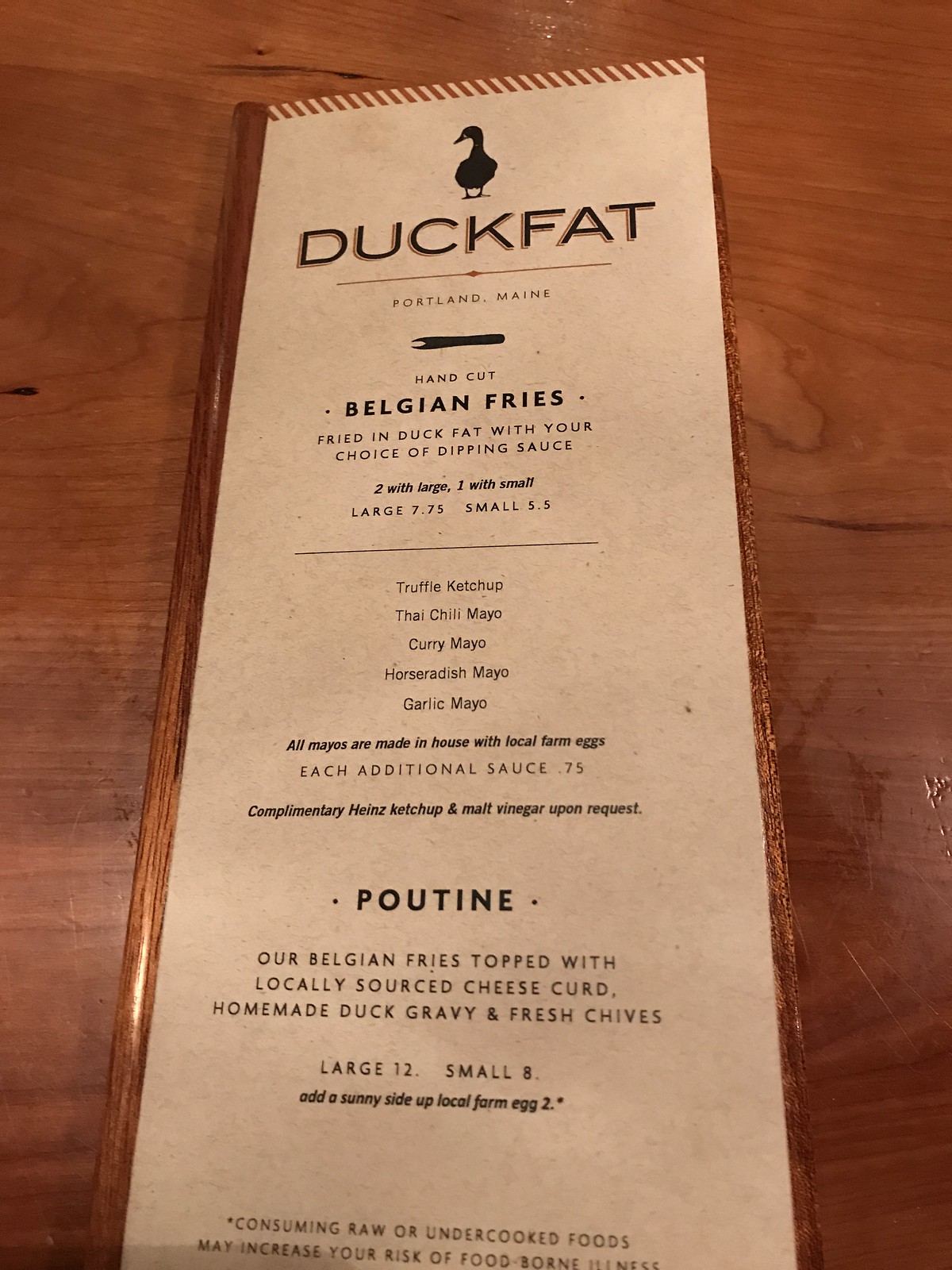The image depicts a menu placed on a wooden table at the restaurant "Duck Fat" in Portland, Maine. The menu itself features a wooden border, giving it a rustic appearance. At the top of the menu is a silhouette of a duck looking to the left, symbolizing the restaurant's name. 

The menu, printed on light beige paper, details the offerings in clear, legible text. It begins with a section titled "Hand Cut Belgian Fries," which are fried in duck fat. Patrons can choose from a variety of dipping sauces, listed as truffle ketchup, Thai chili mayo, curry mayo, horseradish mayo, and garlic mayo. These mayos are made in-house using local farm eggs. Complimentary Heinz ketchup and malt vinegar are available upon request. The prices for the fries are specified as $7.75 for a large and $5.50 for a small portion.

A faint horizontal line separates this section from the next, which is titled "Poutine" in bold black letters. The description for poutine highlights Belgian fries topped with locally sourced cheese curd, homemade duck gravy, and fresh chives. The prices for poutine are listed as $12.00 for a large serving and $8.00 for a small serving.